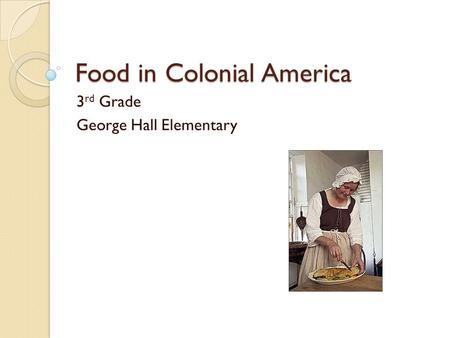**Food in Colonial America**

*Third Grade  
George Hall Elementary*

The web page, presumably from a school yearbook, features a centered title in dark brown text, reading "Food in Colonial America." Below this main heading, the subheadings "Third Grade" and "George Hall Elementary" are also centered. To the left, a pale border, described as bone-colored or very faded pink, runs down the page. This border includes decorative elements such as a blue dot, a yellow dot, and a semicircle resembling a bookmark.

To the lower right of the page, an image depicts a woman dressed in 18th-century colonial attire. She wears a white bonnet and a dress with a dark brown top and light bone-colored bottom. The woman appears to be in a kitchen, evidenced by visible tables and windows in the background. She is engaged in the act of cutting a large pie or sandwich on a tray, likely with a knife, preparing to serve it.